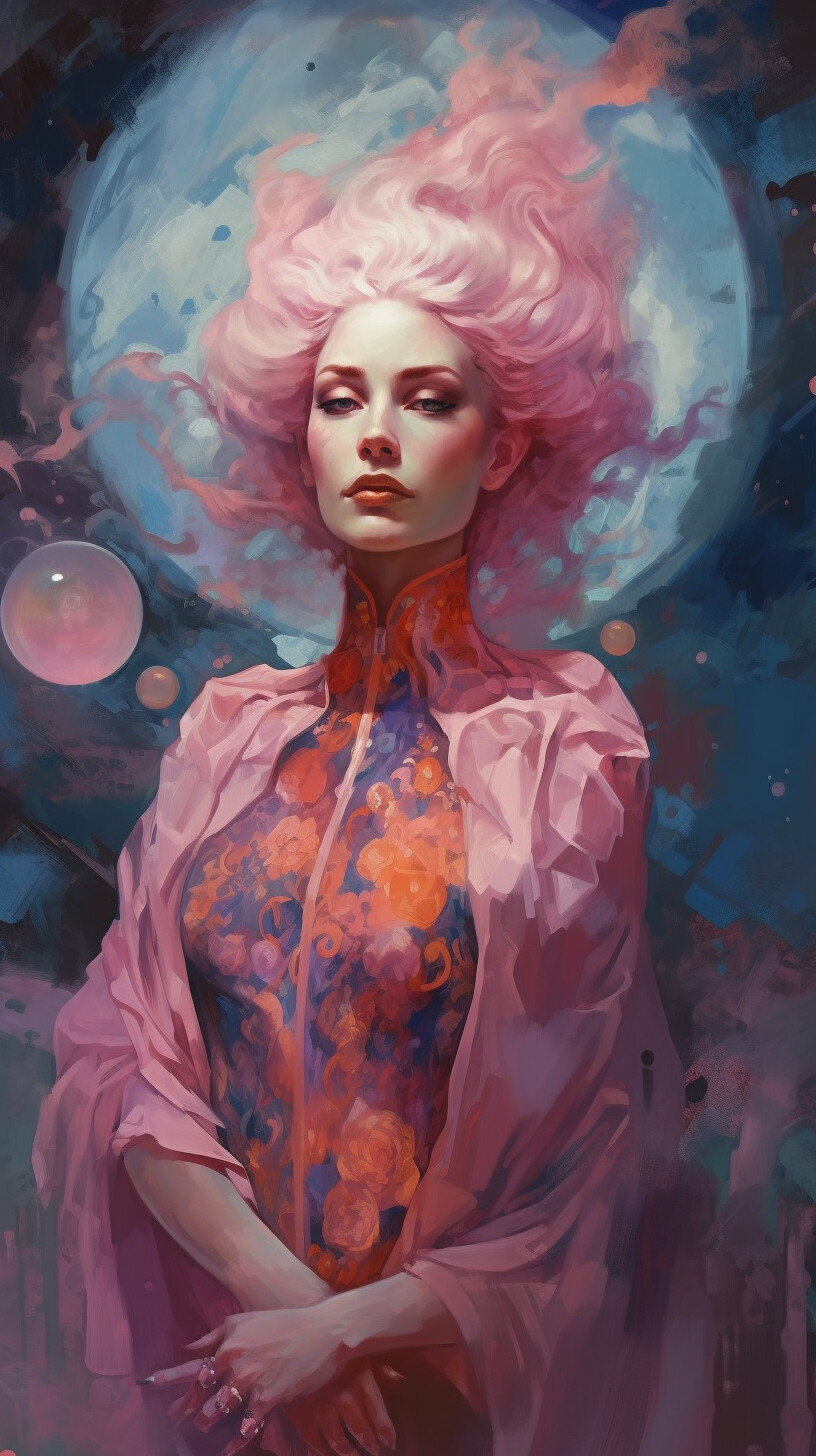The image is a detailed digital painting of a young Caucasian woman with long pink hair that appears to be flowing upward as if caught in a breeze or underwater current. She has red lipstick, light brown eyebrows, classic facial features, and a graceful long neck. Her attire includes a pink shawl draped over her shoulders and a zip-up dress adorned with a multicolored floral pattern in shades of orange, pink, blue, and purple, featuring a high collar. Her arms are positioned in front of her waist with her left hand over her right, displaying rings on her fingers. The background consists of a large, bluish-white moon directly behind her head against a dark blue, nighttime sky. Adding a whimsical touch, pink bubbles float through the air around her. The woman's serene expression and detailed depiction suggest a portrayal of a fantasy goddess or nymph, standing prominently as the central figure in this ethereal artwork.